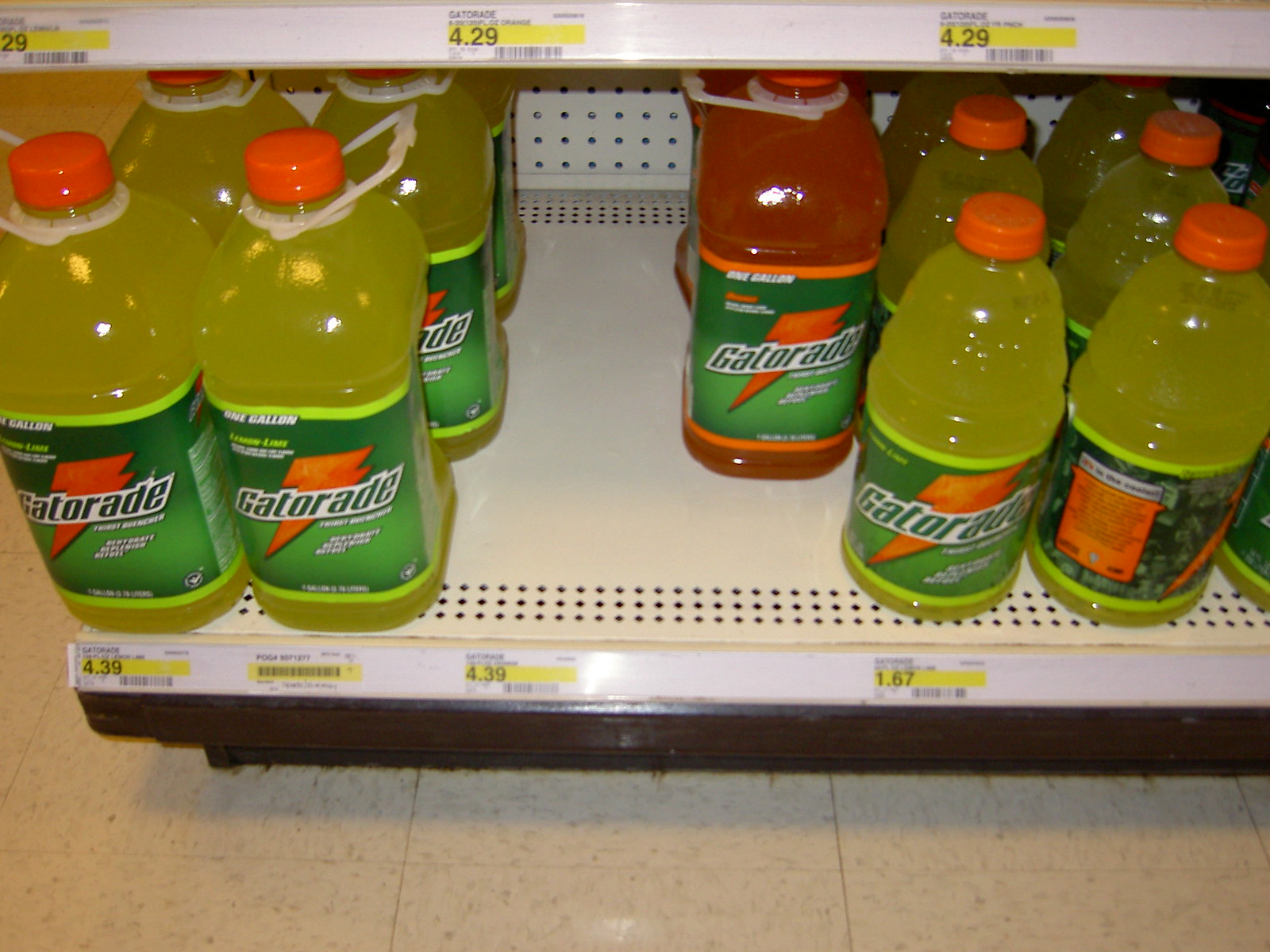In the image, an assortment of Gatorade bottles is displayed on supermarket shelves. The bottles are arranged by size and flavor, with larger variants positioned above the smaller ones. The flavors include a vibrant yellow and a bold red, available in different sizes.

The larger bottles, likely 1 liter in volume, feature an ergonomic handle for convenient carrying, while the smaller, approximately half-liter bottles, lack this feature. Each bottle is adorned with a distinctive green label that covers roughly three-quarters of the bottle's height, terminating about a quarter of the way from the top. This label prominently displays the "Gatorade" brand name, accompanied by an iconic orange thunderbolt logo. Each of these bottles is priced at $4.39, as indicated by the shelf label below them.